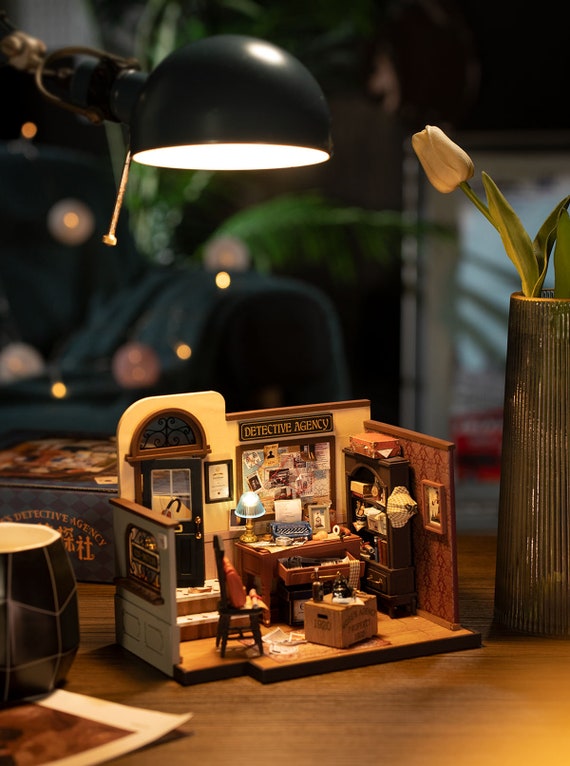The image depicts a realistic photograph of a detailed diorama resting on a brown office desk. The diorama, approximately the size of a girl's dollhouse, represents a scene from a "Detective Agency" office. It features a desk with a lamp and a typewriter, and an open drawer spilling papers and objects. The backdrop of the diorama includes a door with a glass transom window and a sign that reads "Detective Agency." On the right wall, a bookshelf holds various objects, while the floor holds a box with a cup on top. Nearby, a small wooden chair appears to have a bag placed on it. Over the diorama, a suspended black lamp casts light directly onto the scene. Adjacent to the diorama, a brown-and-gold vase contains a single off-white tulip. The real office space around the diorama includes a dark blue couch, a couple of indoor plants, and a large gray mirror leaning against the wall.